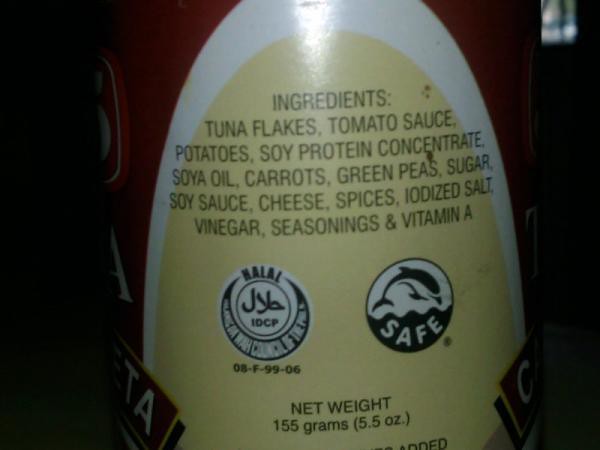The image displays a dark, shadowed photograph of a red can or bottle, viewed from the back. The left and right sides of the image are heavily shadowed, enhancing the prominence of the central label. This label features an oval-shaped tag outlined in white with a yellow interior, presenting a list of ingredients in black text. The ingredients listed are tuna flakes, tomato sauce, potatoes, soy protein concentrate, soy oil, carrots, green peas, sugar, soy sauce, cheese, spices, iodized salt, vinegar, seasonings, and vitamin A. Below the ingredients list are two distinctive circular symbols. The left circle contains text that includes "10CP" and "H-A-L-A-L," likely in a foreign language, and the right circle is white and blue, featuring an image of a blue dolphin with the word "safe." At the bottom of the label, the net weight is specified as 155 grams or 5.5 ounces. The can is positioned on a table against a black background.